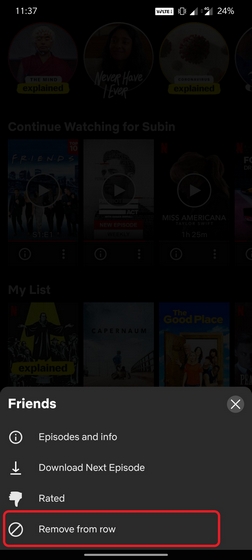This is a detailed screenshot from a movie streaming service interface, primarily dark in color with prominent yellow accents. The screen is dimmed because a friends interface has been activated at the bottom of the page.

In the dimmed section at the top, the interface shows various lists for the profile named "Subin." From what is visible, the top list is labeled "Continue Watching for Subin,” followed by another list titled "My List," which contains a collection of movies and shows. Above these lists are suggested movies, partially visible.

The friends interface, located at the bottom, is clearly labeled "Friends" at the top. To the right of this label is a small "X" symbol for closing the interface. Below the "Friends" label are four interactive options:
1. An eye symbol with the label "Episodes and Info."
2. A download symbol with the label "Download Next Episode."
3. A thumbs-down symbol labeled "Rated."
4. A circle with a diagonal slash, labeled "Remove from Row," which is highlighted with a red rectangle outline, indicating it has been selected or is currently active.

This image appears to be an edited screenshot, modified to showcase the "Remove from Row" option distinctly.